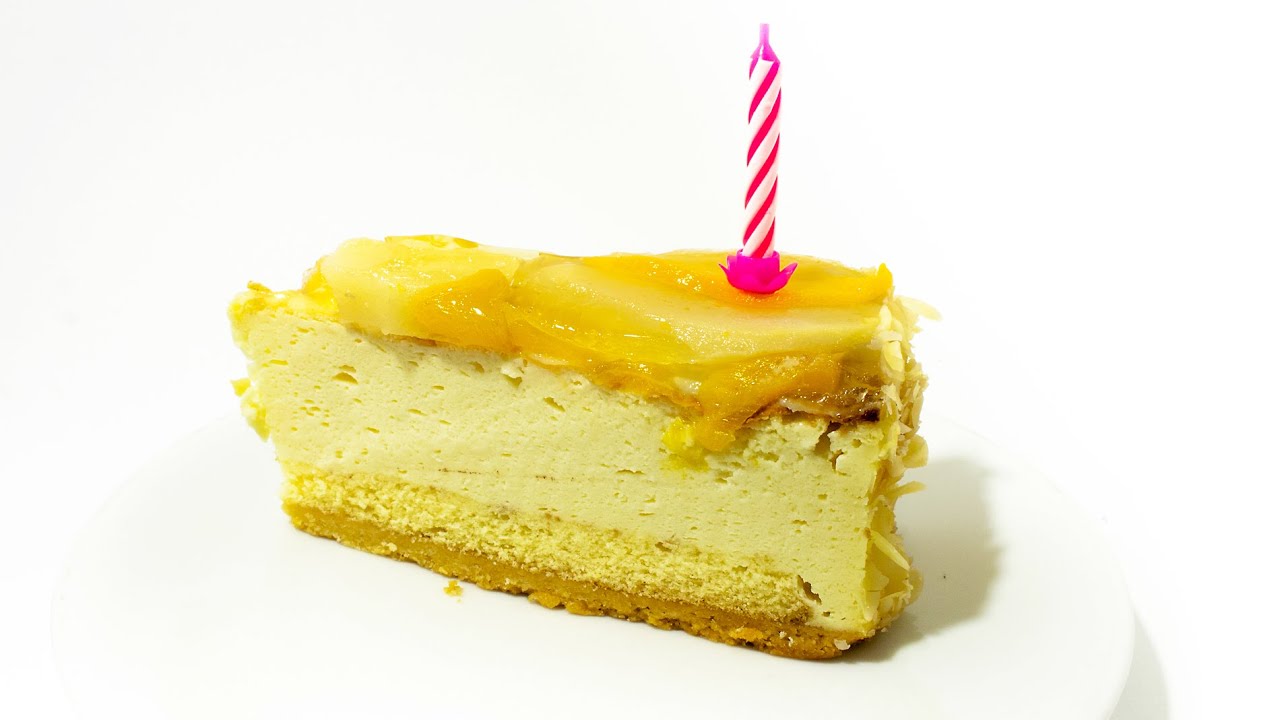This is an image of a piece of lemon meringue pie on a white plate, set against a completely white background. The photograph, likely taken in a studio with artificial lighting from the left, captures the pie's shadow falling to the right. The pie comprises multiple layers: a graham cracker crust at the bottom, a fluffy and airy sponge layer, a creamy and thick cheesecake-like filling, and a runny, custardy lemon topping that adds an inviting shine. Atop the pie is a pink and white striped birthday candle, suggesting a celebratory occasion. The point of the pie is oriented to the left of the image, and the overall appearance showcases various shades of yellow, enhancing the detailing and texture of the dessert.